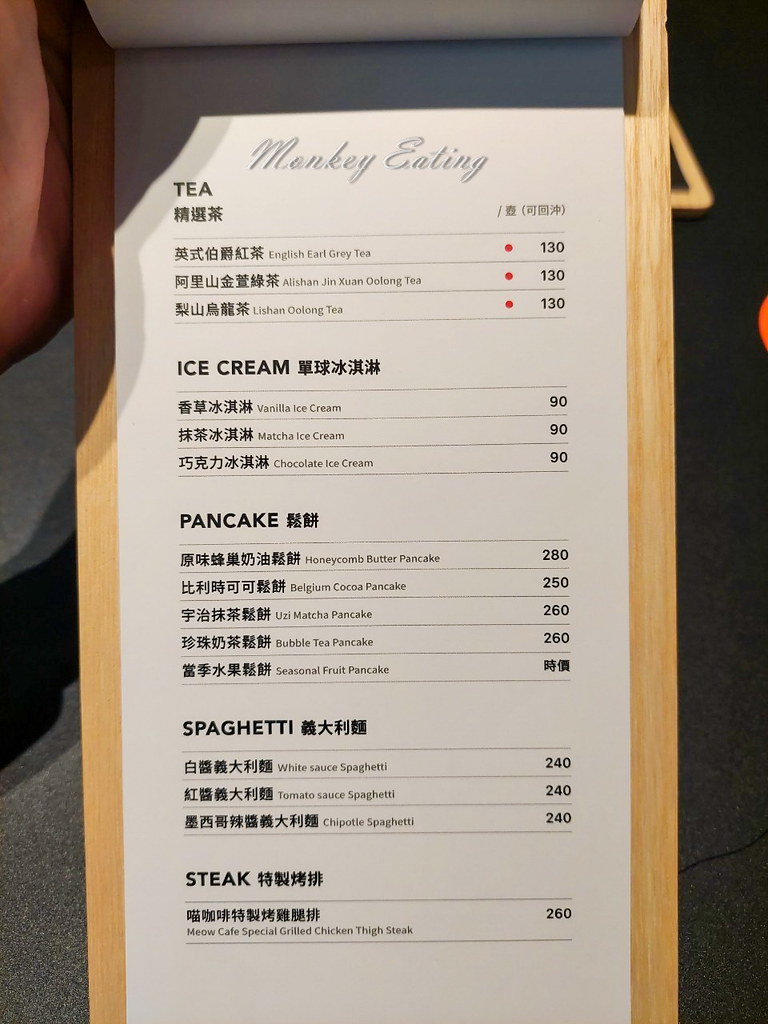A detailed descriptive caption:

The image features a restaurant menu presented elegantly inside a bamboo box. The menu, held up by a hand in the top left corner, showcases a stylish blend of script and block text. At the top, a script font reads "Monkey Eating," followed by the phrase "Tea" in a straightforward sans-serif font, accompanied by Chinese characters. The right side of the menu also contains more Chinese text. The tea section lists several items, each introduced by Chinese characters and followed in English: "Tea, Earl Grey Tea - 130," "Hao Shan Jin Xuan Oolong Tea - 130," and "Lishan Oolong Tea - 130." Following the tea section, the menu prominently displays an "Ice Cream" section in bold, featuring "Vanilla Ice Cream - 90," "Matcha Ice Cream - 90," and "Chocolate Ice Cream - 90." Below these, there are sections labeled "Pancake Menu" and "Spaghetti Menu" in large fonts. At the bottom, under the "Steak Menu" section, is a single item: "Miao Cafe Special Grilled Chicken Thigh Steak - 260."